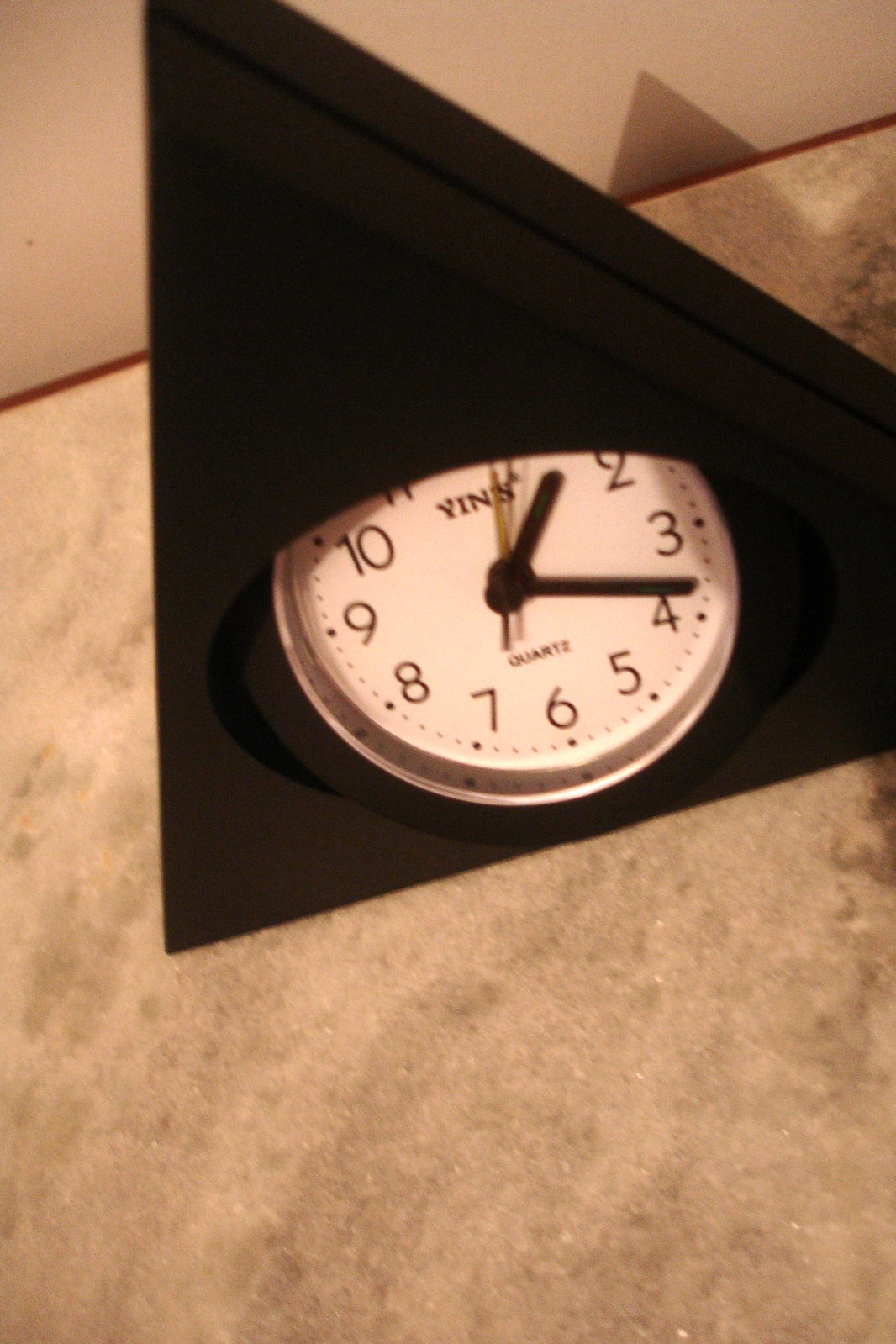This close-up image features a triangular clock encased in a sleek black cabinet. The clock face is off-white and bordered with a silver trim. The dial displays dark brown numerals from 1 to 12, providing a stark contrast against the light background. Prominently marked at the bottom of the clock face is the word "Quartz" in dark brown lettering. The time is indicated by thick dark brown hour and minute hands, accompanied by a thin, light brown second hand. Inscribed at the top of the clock face is the brand name "Y-I-N-S." The clock is positioned centrally on a beige marble countertop, which reflects the clock and adds a sense of depth to the image. The backdrop features a beige wall, enhancing the overall neutral and sophisticated color palette of the scene.